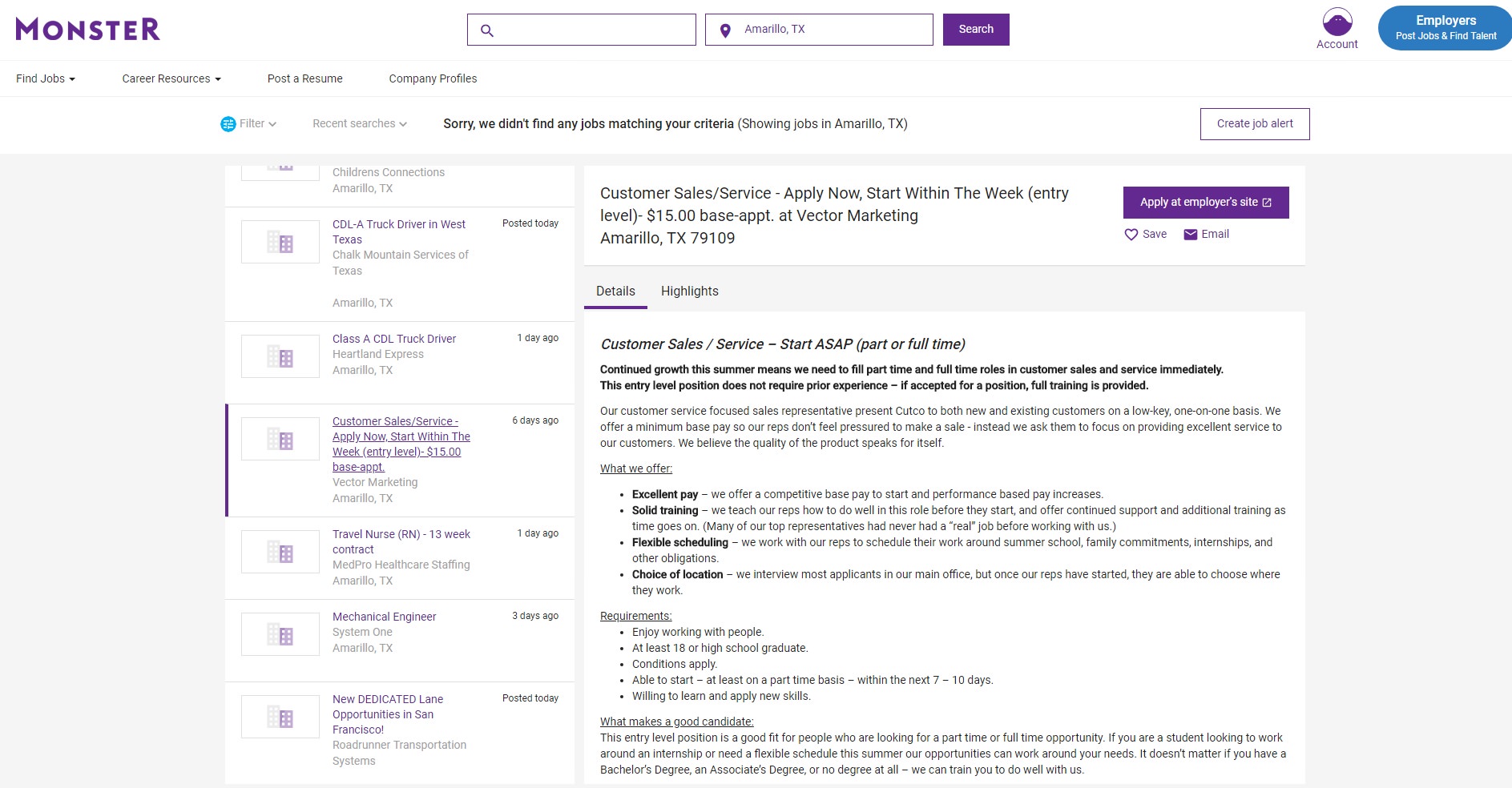This screenshot showcases the Monster job search website, highlighting its user-friendly interface that offers various functionalities. At the top, there are intuitive buttons for finding jobs, accessing career resources, posting a resume, viewing company profiles, and searching for specific criteria. A location filter is set to Amarillo, Texas, displaying job listings relevant to this area.

The listed jobs include positions such as CDL-A Truck Driver in West Texas, CDL-A Class A Truck Driver, Customer Sales, Travel Nurse, Mechanical Engineer, and new dedicated lane opportunities in San Francisco. The screenshot captures a job listing for a Customer Sales/Service role with Vector Marketing, which offers a $15 base rate per appointment.

Detailed information about this job is visible, specifying that it is a Customer Service-focused Sales Representative position for Cutco. The job can start immediately and is available both part-time and full-time. Additional highlights include excellent pay, solid training, flexible scheduling, and location choices. The screenshot also details job requirements and characteristics of an ideal candidate, with a button leading to the employer’s website for application.